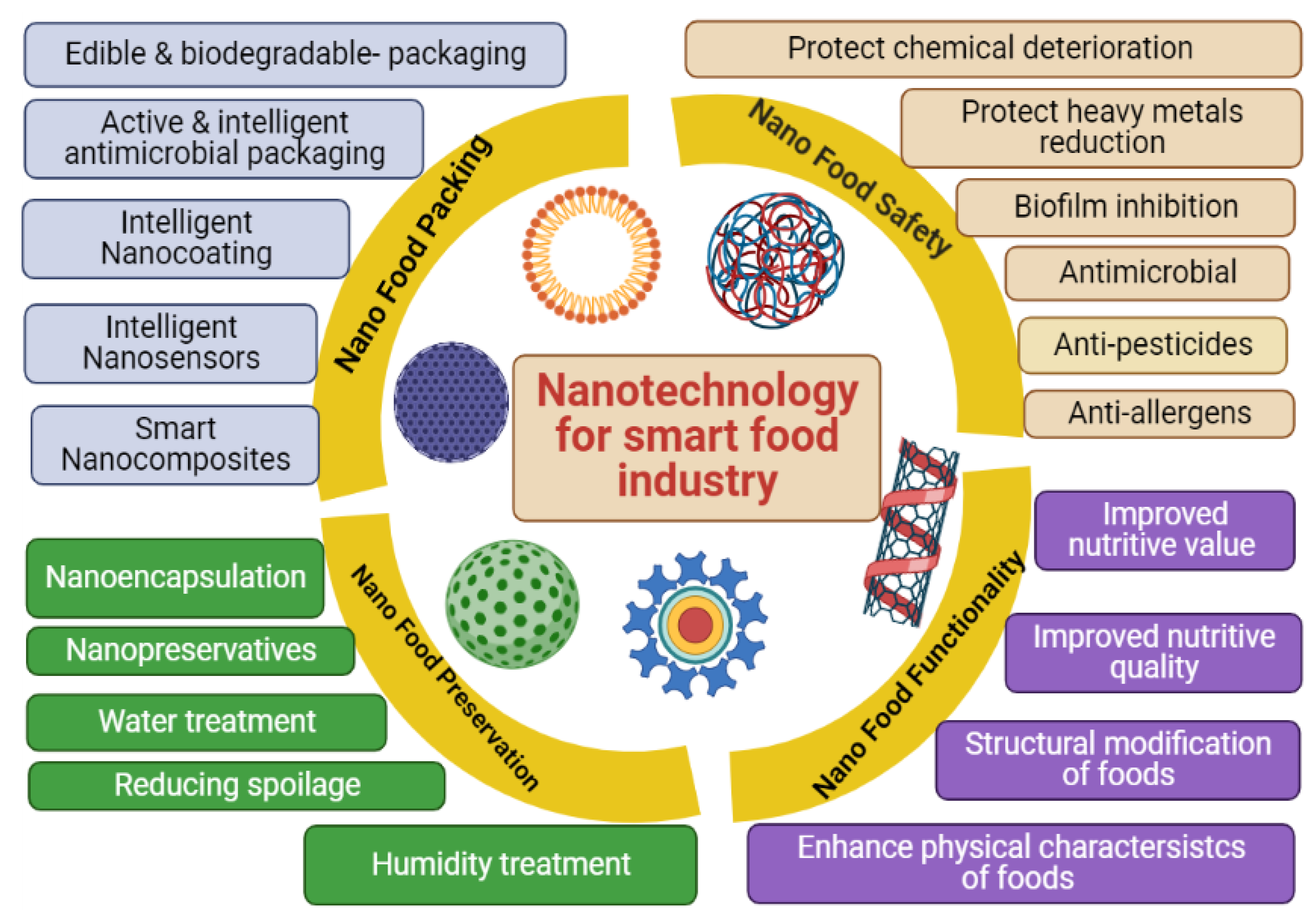This detailed infographic on "Nanotechnology for Smart Food Industry" is centered around a small rectangular box with red text highlighting the central theme. Encircling this central box are various scientific symbols and molecular structures, including interlocking red and blue circles, a hexagonal ribbon, concentric circles, and dotted spheres in blue, green, purple, and red, symbolizing different aspects of nanotechnology applications.

Surrounding the central theme, a yellow circle is divided into four quadrants, each emphasizing a key area of nanotechnology: Nanofood Packaging (top left), Nanofood Safety (top right), Nanofood Preservation (bottom left), and Nanofood Functionality (bottom right). Each quadrant is supported by rectangular boxes with more specific details.

In the upper left, blue boxes list: Edible and Biodegradable Packaging, Active and Intelligent Antimicrobial Packaging, Intelligent Nano-coating, Intelligent Nanosensors, and Smart Nanocomposites. The bottom left features green boxes with: Nano-encapsulation, Nanopreservatives, Water Treatment, Reducing Spoilage, and Humidity Treatment.

In the upper right, tan boxes cover: Protect Chemical Deterioration, Protect Heavy Metals Reduction, Biofilm Inhibition, Antimicrobial, Anti-pesticides, and Anti-allergens. The bottom right, highlighted in purple boxes, includes: Improved Nutritive Value, Improved Nutritive Quality, Structural Modification of Foods, and Enhanced Physical Characteristics of Foods.

Visually, the graphic combines educational content with a vivid color scheme and symbols to elaborate on the roles and applications of nanotechnology in the smart food industry, making it an informative and engaging piece possibly used for educational purposes or employee training.